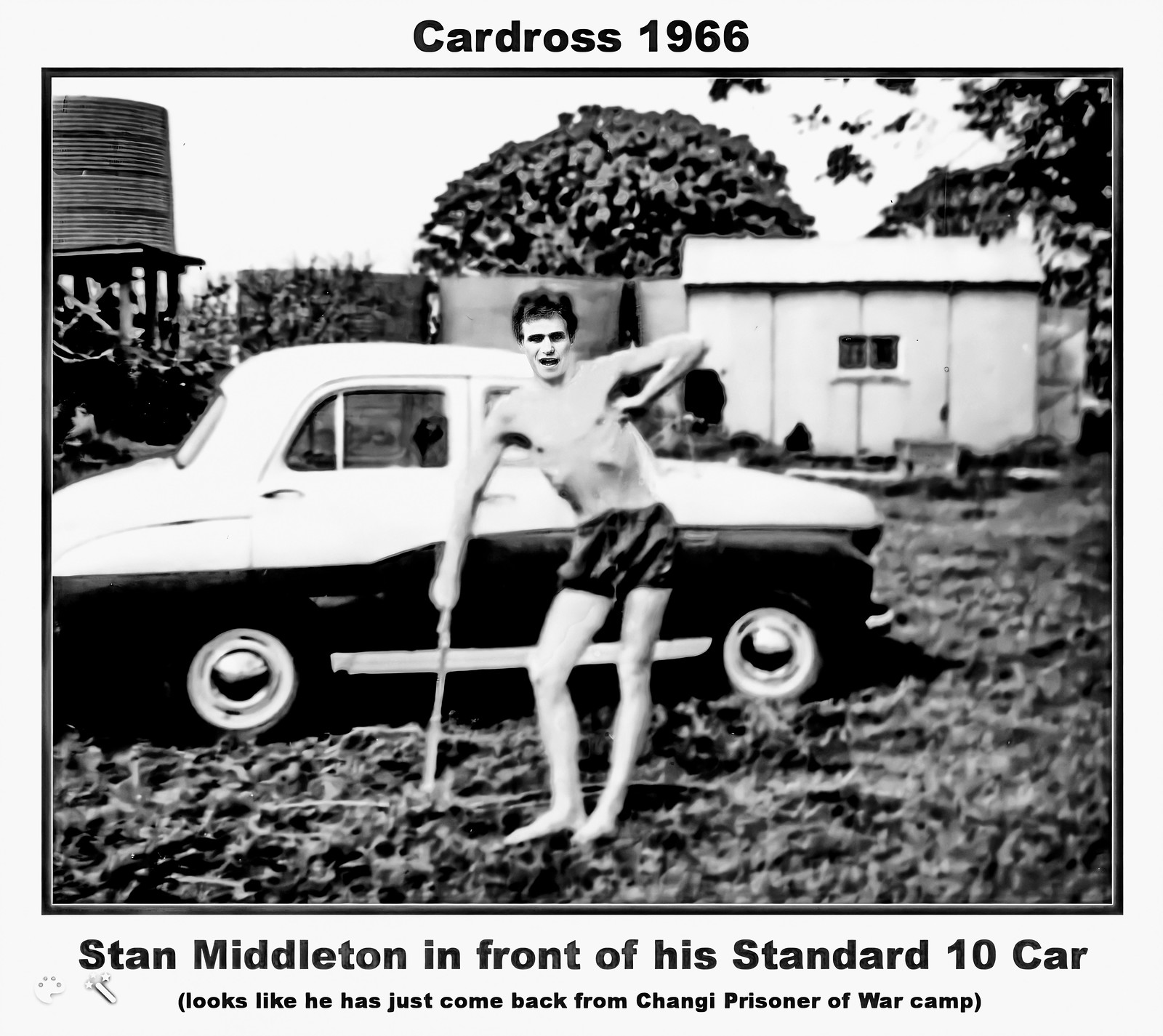This black-and-white photograph, taken outdoors during the day, features an extremely thin young white man standing barefoot and shirtless, wearing only a pair of shorts. His emaciated frame reveals visible ribs, and his right hand leans on a stick for support while his left hand is tucked under his armpit. The man, identified in the text as Stan Middleton, stands in front of a two-tone, 1950s-style, two-door sedan, known as a Standard 10. The text on the photograph reads, "Car Dross 1966," with a caption below stating, "Stan Middleton in front of his Standard 10 car." In smaller text beneath, it suggests, "Looks like he has just come back from Changi prisoner of war camp." The background reveals a rustic setting with a gabled shed, a water storage tank, three large cylinders, and a tree. The ground beneath him seems cluttered with debris like leaves and weeds, adding to the raw, historical ambiance of the scene.